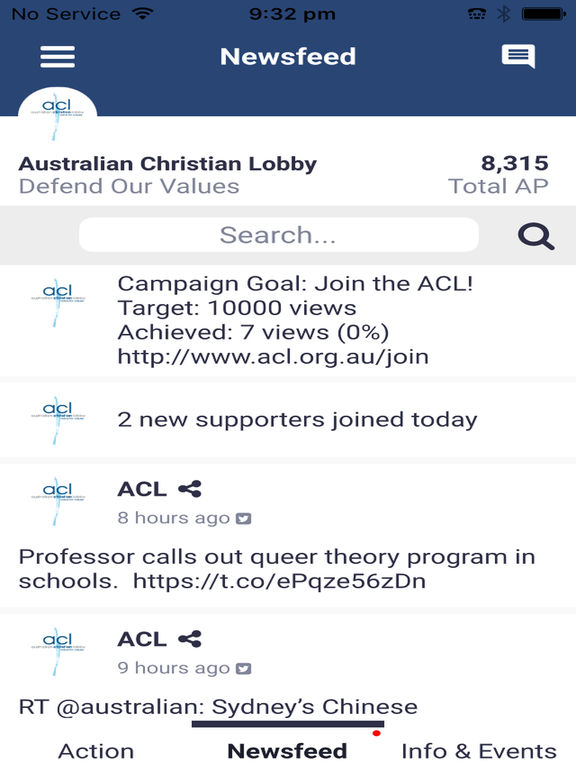This is a detailed screenshot of a newsfeed application affiliated with the Australian Christian Lobby (ACL). At the top, the status bar indicates "No Service" but shows strong Wi-Fi connectivity at 9:32 p.m. In the status row, there is also a visible icon of a phone on a keyboard, yet its function is unclear. Additionally, there's a receiver icon resting on a brick-like design, alongside standard indicators such as a Bluetooth icon, a full battery meter, and a hamburger menu on the left.

The main interface features a title bar with a white background and a medium desaturated blue overlay. On the left side, a speech bubble icon with three lines inside denotes notifications or messages. Prominently displayed is the ACL logo cascading into both the title bar and the central content area, accompanied by bold text reading "Defend Our Values."

To the right of this, there is an intriguing figure, "8,515 Total AP," but its exact significance remains unclear. Below, a search bar invites users to explore content by typing keywords. The newsfeed itself consists of several entries, each marked with a distinctive logo and headline.

The first newsfeed item announces a campaign goal: "Join the ACL, Target: 10,000 views, Achieved: 7 views (0%)." A link to join accompanies this entry. The following entry notes, "Two new supporters joined today," again marked by a relevant logo.

Continuing down, another update, timestamped eight hours ago, has the ACL logo and a share link. The headline states, "Professor calls out queer theory program in schools," with an embedded link for further reading.

The next item showcases the ACL logo with a share option, timestamped nine hours ago. Following this, a brief and cryptic note reads "RT Add Australian, Sydney’s, Chinese," which might imply a retweet or repost.

At the very bottom of the feed, a navigation bar presents options for "Action," "Newsfeed," and "Info and Events." The "Newsfeed" tab is currently active, delineated by bold and darker text, indicating that users are viewing the primary updates and information shared by the Australian Christian Lobby.